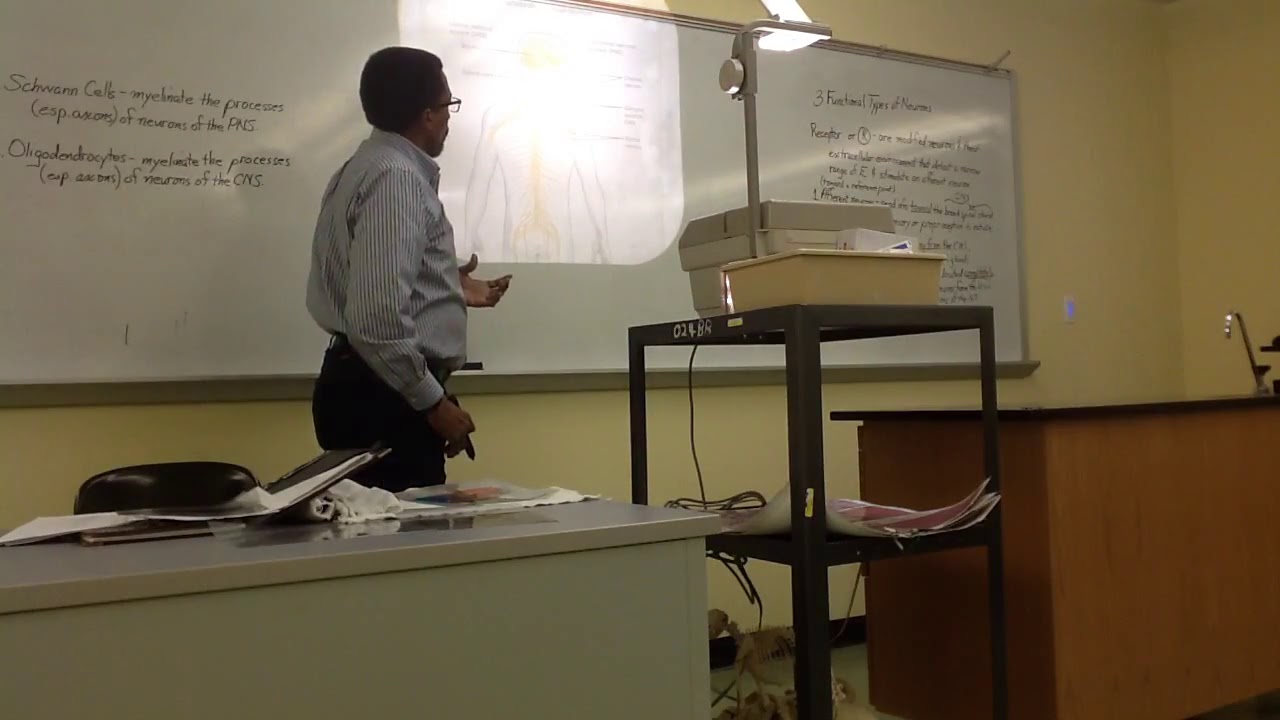In this image, we see an older African-American male professor, wearing glasses, a striped collared shirt, and long pants, engaged in teaching. He stands turned to the side, near two distinct desks. To his left is a white desk with a chair behind it, cluttered with papers. On the right, there is a wooden lecturing podium, slightly higher than the white desk, resembling a science work table complete with a sink and black countertop. Between these two surfaces, there is a classic cream-colored overhead projector, which is projecting an image onto a large whiteboard mounted at the front of the room. The whiteboard has writing on both the left and right sides, although the specifics of the text are difficult to discern. The scene is set indoors, likely in a classroom, during the middle of the day, with an array of colors including tan, yellow, gray, black, white, red, pink, and brown adding to the academic atmosphere.